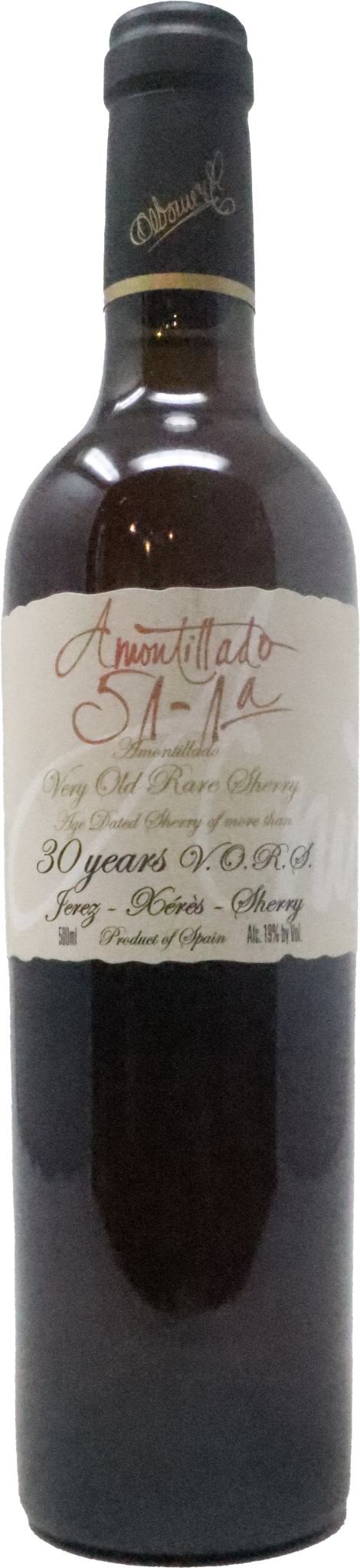This photograph showcases an elegant and striking bottle of Amontillado sherry, aged for 30 years. The bottle itself is made of dark, almost black glass that reflects light and surrounding objects, creating a dramatic visual effect. The top of the bottle features a black and gold seal that must be broken to open the bottle, emphasizing its premium quality. The label is a tan color with the name "Amontillado 5A-A" prominently displayed in red cursive letters. Below this, additional descriptive text is printed in black. This bottle exudes a sense of sophistication and suggests that it is a valuable and well-aged libation.